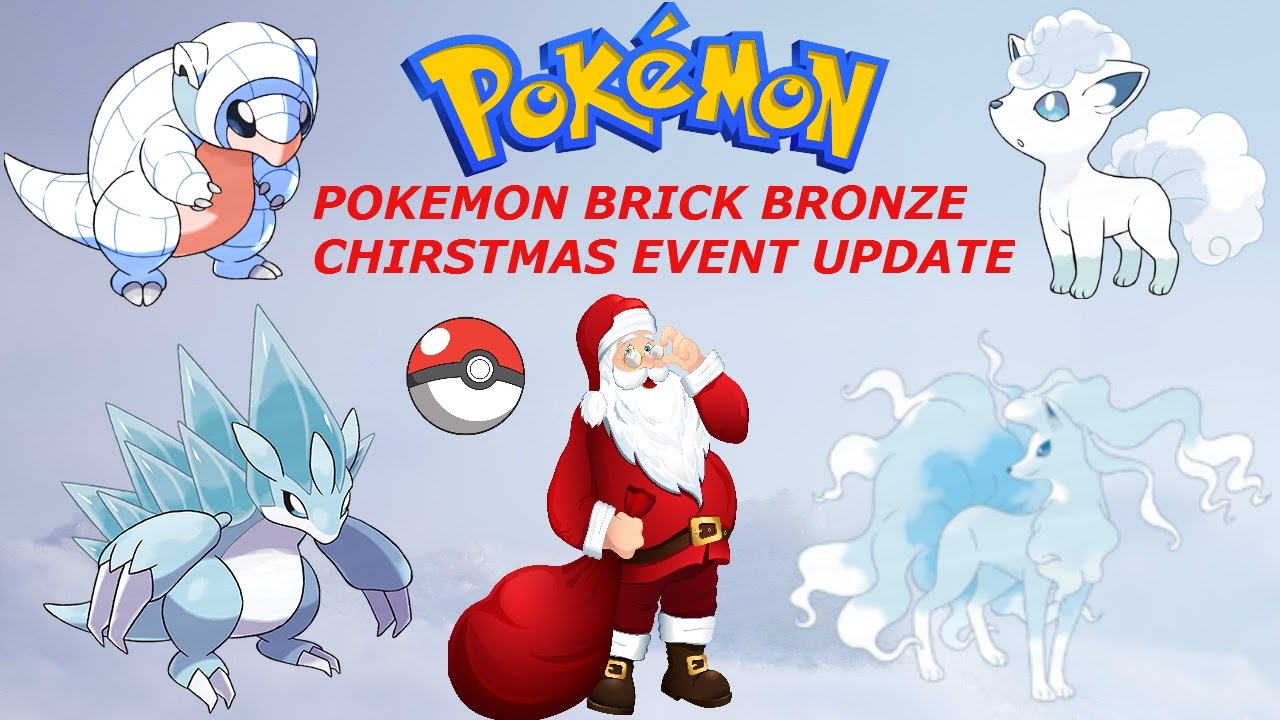In this vividly crafted image, we are presented with a promotional visual for a Pokemon event, specifically highlighting a Pokemon Brick Bronze Christmas update. The background is a gradient of various lavender shades, transitioning from the lightest hues in the lower corners and bottom to the darkest shade in the upper left corner, creating a serene yet dynamic backdrop.

At the center of the image, the phrase "Pokemon Brick Bronze Christmas Event Update" is prominently displayed in bold, eye-catching red text. Above this text, the iconic Pokemon logo stands out in its classic yellow, with letters outlined in blue, giving it a striking three-dimensional appearance that captures the essence of the beloved franchise.

In the upper left corner, a charming character resembling an armadillo is depicted. This character is predominantly white, with a distinctive pink chest, small ears, and a pointy tail, standing upright on its two back legs, adding a touch of whimsy to the scene. Directly below this character, there is an imposing dragon-like figure rendered in shades of blue and white. This creature has its arms extended to the sides, each foot adorned with two long talons, and a spiky back, exuding a sense of power and elegance.

Dominating the central area of the image is a jolly depiction of Santa Claus. He stands prominently, holding a large red sack, symbolizing the festive spirit of the Christmas event. Santa's presence adds a warm and inviting touch to the promotional material, tying together the theme of the holiday update in the Pokemon Brick Bronze game.